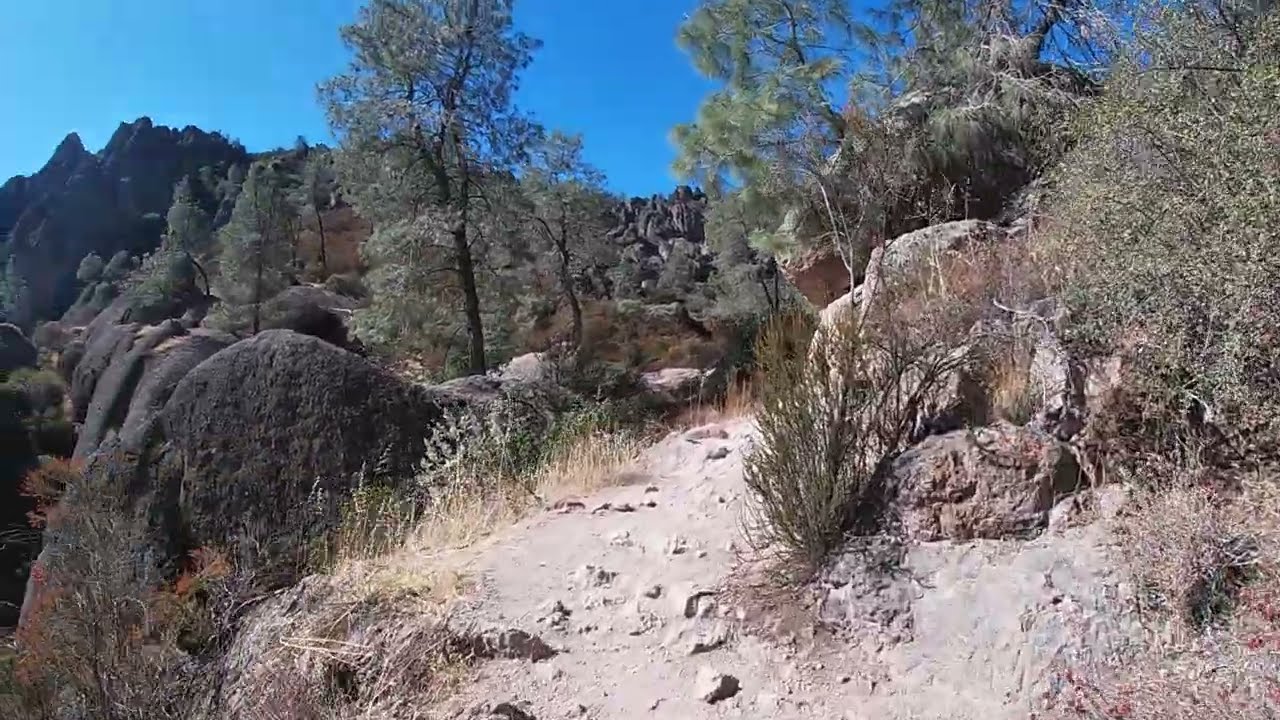The image shows a high desert walking trail surrounded by a mixture of pale green and dry-looking shrubbery and rustic boulders, both gray and pale brown. Dominating the left side of the scene is a full-grown tree with a backdrop of rocky ledges and distant mountains. The sandy path, light beige in color, weaves through an uneven terrain dotted with clusters of bushes and both large and small boulders. Cliffs and rounded hills frame the scene, their gray tones contrasting with the vibrant blue daytime sky above. The landscape appears very dry and deserted, with no people or buildings in sight, evoking a sense of isolation and serene wilderness. The arid climate hints that this could be somewhere in Colorado, Wyoming, or possibly Utah.